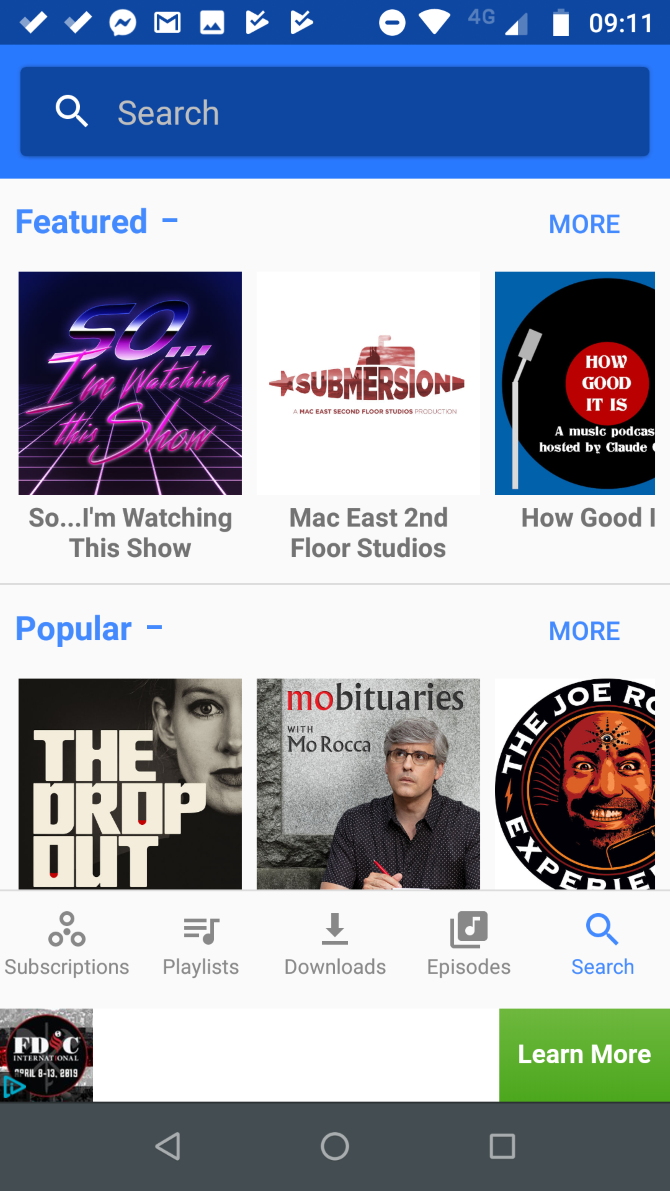This image captures a cell phone screen displaying a multimedia application interface. At the top of the screen, a row of icons is visible, including check mark icons, a messenger icon, a Google Mail icon, a pictures icon, and triangle icons with check marks in the middle. The upper part of the screen is blue, featuring a 4G signal indicator, a battery icon, and the time displayed as 09:11.

Beneath this, there is a blue search bar. Below the search bar, the main section of the screen is categorized into "Featured" content. The first featured item is an image reminiscent of the 90s, with text stating, “So... I’m watching this show.” The second featured item is a stylized image with the text "Submerge In" resembling a submarine graphic, labelled "Mac East Second Floor Studios.” The third icon, somewhat cut off on the right, depicts a record and includes the text, “How Good It Is,” a music podcast hosted by Claude.

Further down, there is a section titled "Popular" in blue. Here, one image is titled "The Dropout," featuring the face of a Caucasian woman. Another image depicts "Mobituaries with Mo Rocca," followed by the image for "The Joe Rogan Experience."

At the bottom of the screen, a navigation bar includes various buttons: Subscriptions, Playlists, Downloads, Episodes, and a search icon, providing multiple ways to browse and manage media content on the application.